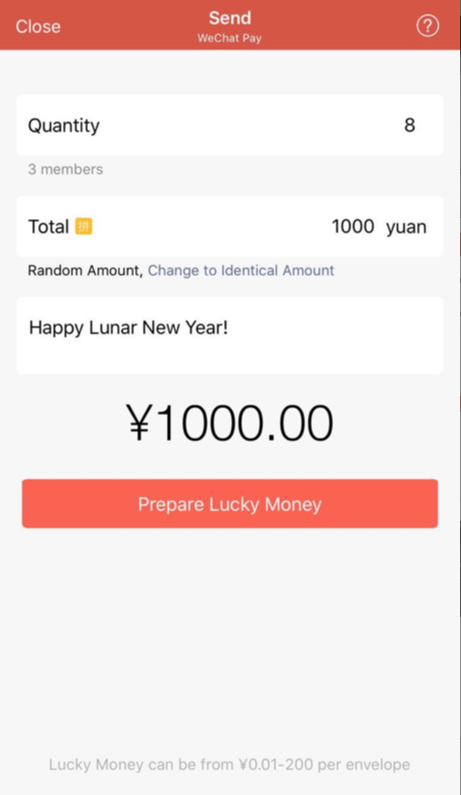**Detailed Caption for WeChat Pay Screen:**

The WeChat Pay interface features an orange bar at the top with "Close" on the left, a question mark icon on the right, and "Send" in the center. Below this bar, the header "WeChat Pay" is displayed, indicating that the user is engaged in a payment process. The quantity indicated is eight, divided among three members. The total amount is shown within a yellow box containing a Chinese character, followed by the text "1,000 yuan."

Next to this, in black text, it states "random amount," with an option in lighter gray text to "change to identical amount." Beneath these details, the festive greeting "Happy Lunar New Year!" is prominently displayed with an exclamation point.

Further down, the currency symbol for yuan (¥) is shown next to the specific amount "1,000.00." Below this, a full-width peach-colored button invites the user to "Prepare Lucky Money."

At the bottom of the screen, light gray text informs users that "Lucky Money can be from 0.01 to 200 per envelope." A single black pixel line runs down the entire right edge of the screen capture. The overall background is white, providing a clean and simple visual design.